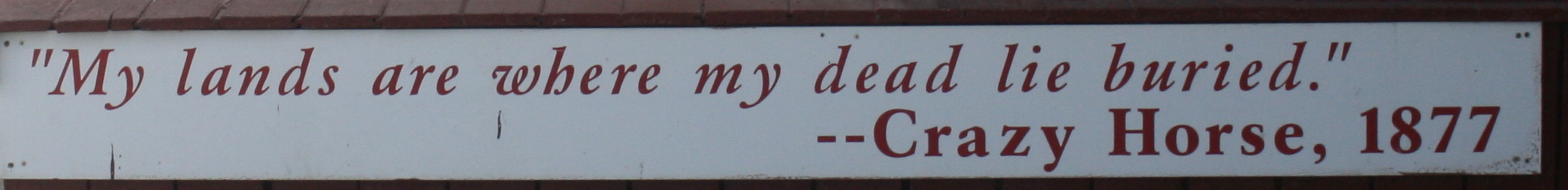The photograph captures a close-up of a rectangular white sign, significantly wider than it is tall, with noticeable damage or corrosion affecting its surface. A quote is prominently featured on the sign in dark red, italicized lettering: "My lands are where my dead lie buried." Below the quote, the source is cited in bolded font: "-- Crazy Horse, 1877." The sign is bordered by a brown edge, and each corner is marked by pairs of small dots. In the background, from the upper left to the center, a wooden plank surface is visible, suggesting the sign might be affixed to or leaning against it. The entire scene is set against a uniformly white backdrop.